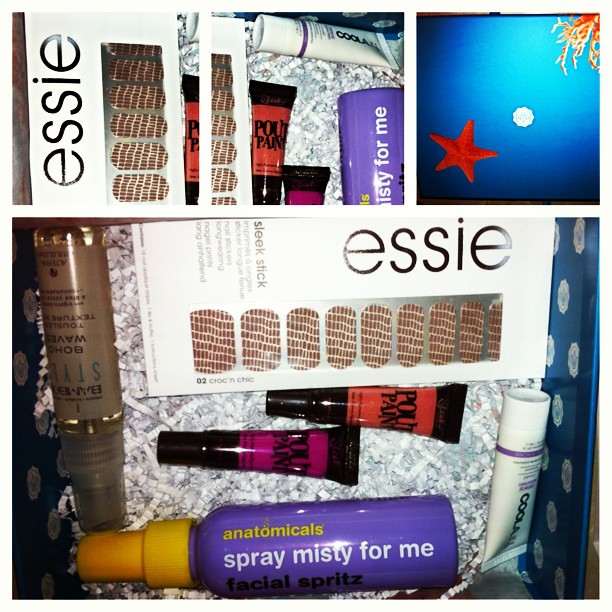This detailed image collage showcases a gift box filled with assorted toiletries and beauty products. The primary photo, situated in the lower section, presents an array of items nestled within shredded paper for cushion. Central to the arrangement is a white box with black text vertically spelling “ESSIO.” Beside it are tubes of various products, including a vibrant red and black tube labeled "Cool Lab," a white tube, and a purple tube with white text saying "Spray Misty for me," which is an anti-anatomical spray with a yellow cap. 

Additional items include a lotion in a brown bottle and several tubes of lip products in shades of pink and red. The photograph on the upper left corner offers a similar view of the box, reiterating the "ESSIO" box and the visible tubes. Meanwhile, the upper right corner features a close-up image of an abstract graphic design with a red star and white circle centered within a blue square, adorned with red plant-like elements in the corner. This collage cohesively displays the diverse range of beauty and skincare products, all elegantly arranged within a gift box setting.